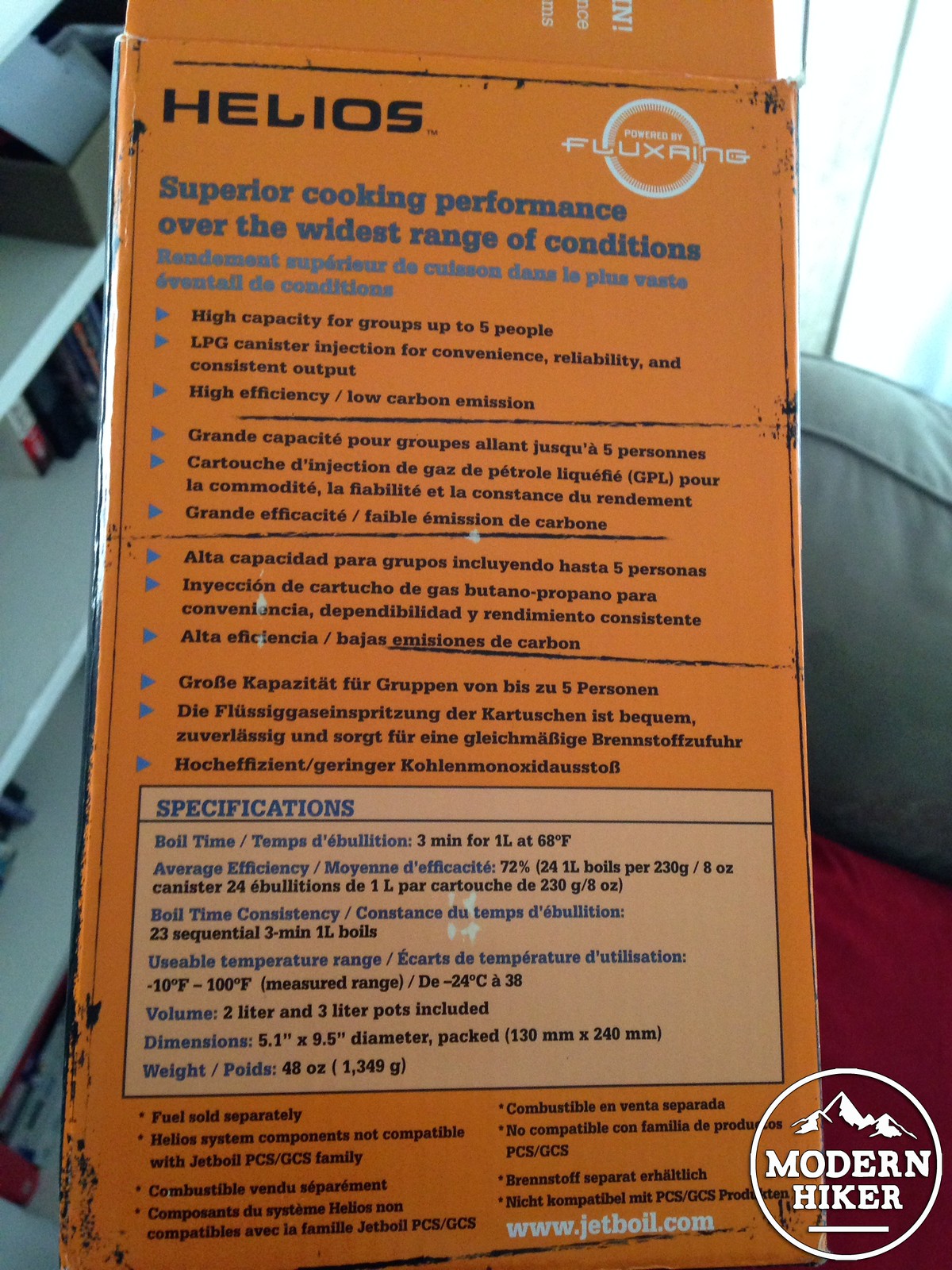This image showcases an indoor setting featuring a gray stairway with a few visible steps leading up. Adjacent to the stairway, the back of a light gray couch is partially visible, adorned with a red cloth draped over it. In the background, a window allows natural light into the space. Prominently displayed in the foreground is an orange package with "Helios" written in bold black lettering. Below this, in blue text, the package claims "superior cooking performance over the widest range of conditions." At the bottom of the package, a small white circle containing a white mountain icon and the words "modern hiker" hint that this product caters to outdoor enthusiasts, likely offering a convenient cooking solution for hikers.